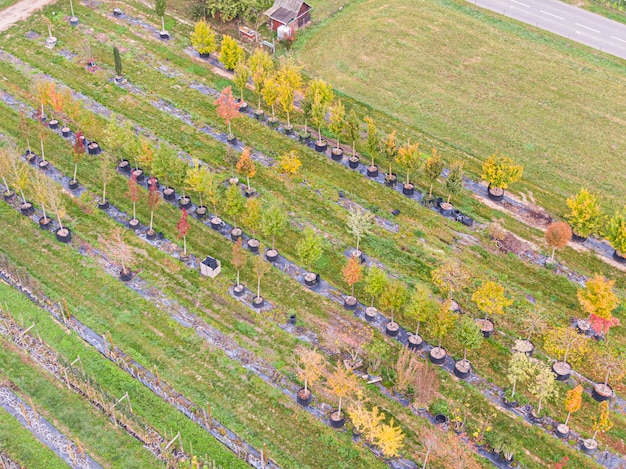This aerial view captures what appears to be a meticulously arranged nursery, possibly a farm, dedicated to cultivating and selling trees and bushes. Central to the image is a barn-like structure in shades of brown and hints of red, positioned next to a neatly mowed grassy area. Extending from the upper part of the photo to the lower right, rows of young saplings—many still in pots—are meticulously organized in linear formations. The trees exhibit a spectacular variety of colors, including vibrant shades of yellow, green, red, pink, and orange, suggesting a rich diversity or possibly a seasonal transition, such as autumn. Patches of bare soil intersperse these rows, enhancing their orderly appearance. The surrounding fields are lush with green grass and are carefully separated. In the upper right corner, a road slices through the landscape, marked with white lines and contributing to the organized layout of the area. The entire scene is soaked in natural hues, with dominant greens, touches of brown, and an array of vibrant tree colors, creating a rich tapestry of rural life from above. The image, possibly a drawing, emphasizes precision and a peaceful rural aesthetic.